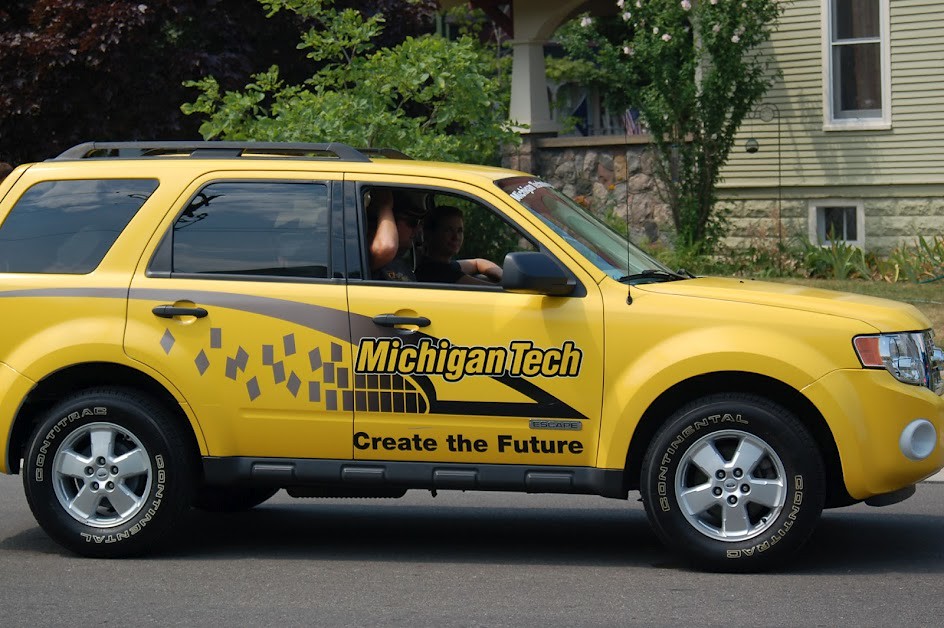This detailed outdoor photograph captures a yellow SUV or crossover vehicle prominently in the frame, with its right side facing the camera. The SUV features a distinctive decorative gray stripe that starts at the back, thickens as it passes through the rear door, and transitions into a black line along the bottom of the front passenger door, accompanied by small black rectangles. Emblazoned along the side are the words "Michigan Tech" in white letters with black trim, followed by "Create the Future" in black text beneath. The SUV is equipped with a black roof rack, and its clean black tires stand out prominently. The right passenger is visible with his arm up and hand resting on his head, while the driver is glancing towards the camera with his left arm propped on the door ledge. The back windows are tinted, obscuring any interior view.

Surrounding the vehicle, a beige house with white trim and a rock wall at the basement level is visible, along with shrubberies and various grasses decorating the nearby area. In the background, trees add a natural element to the scene, complementing the suburban setting. A distinctive antenna extends from the SUV, further adding to the vehicle's character. The overall composition positions the SUV in the majority of the frame, slightly cut off on the left, making it the clear focal point of the image.